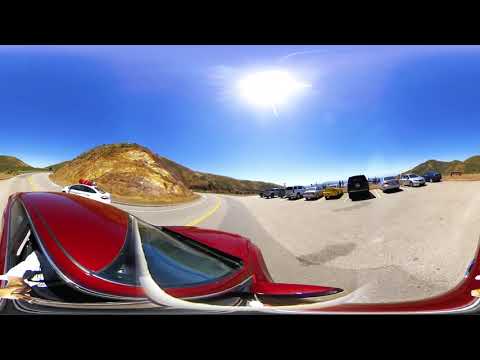The photograph captures a scenic hillside road in Hawaii, adorned with lush greenery and yellow road lines, under a crystal-clear blue sky with bright sunshine. Central to the image is a vibrant red car, suggesting the picture was taken from its side mirror at a unique angle. On the left, the road ascends a hill, providing a sense of upward motion. In the middle of the image, the winding road curves around the hill, framed by an expansive range extending into the distance. 

To the right, a parking lot is visible, filled with various vehicles including a silver van, a black SUV, a yellow sports car, a white pickup truck, and a white Jeep. A striking white car with red luggage on its roof stands out as it travels down the hill road. This scene evokes a sense of adventure and the readiness to embark on a hike, characteristic of an idyllic Hawaiian landscape.